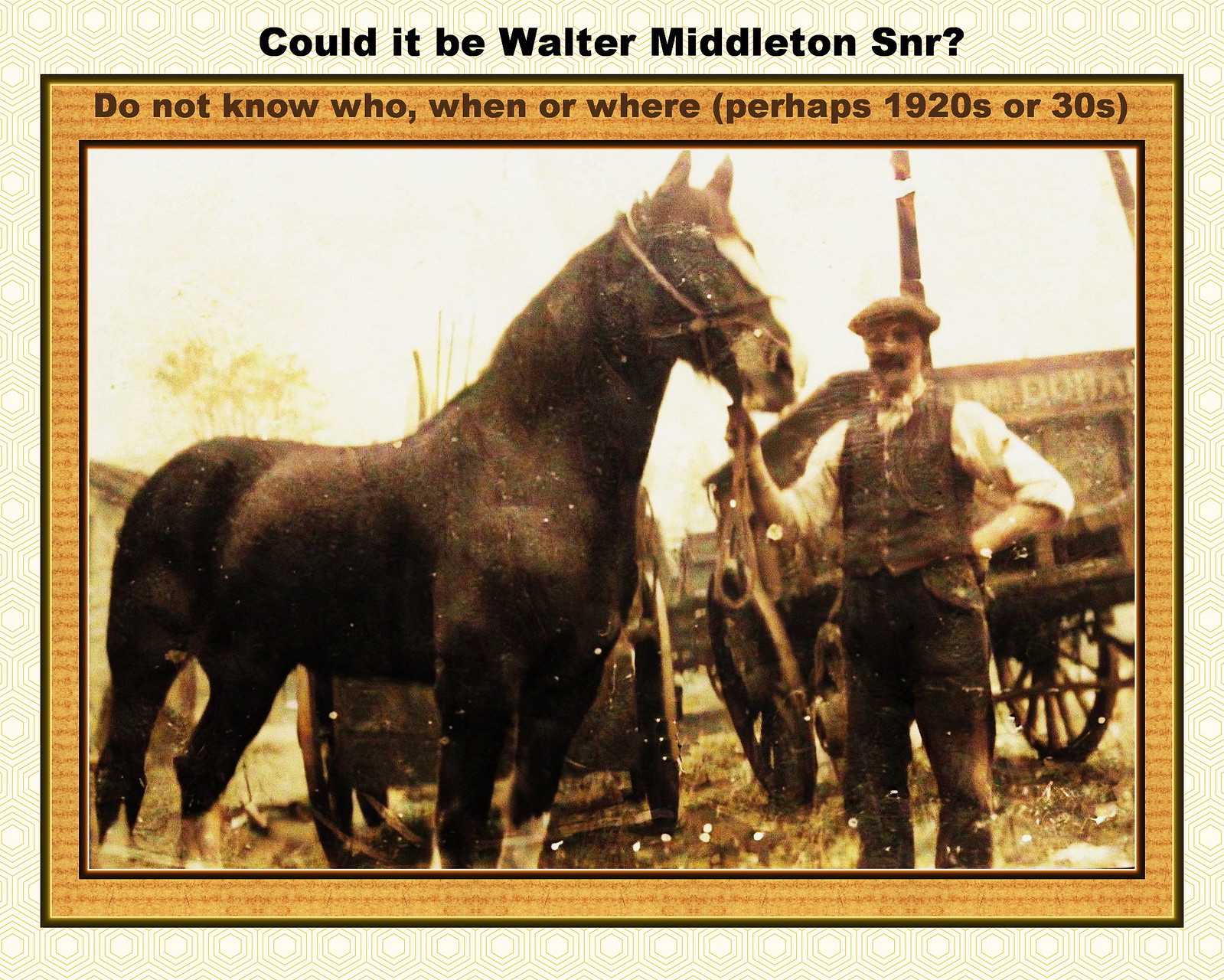This image, reminiscent of a vintage scrapbook or website display, features a sepia-toned, old photograph bordered by an orange frame with a beige background adorned with white hexagonal patterns. At the top of the beige border, in black text, it reads: "Could it be Walter Middleton Senior." Below the image, similar text notes: "Do not know who, when or where (perhaps 1920s or 30s)."

The photograph itself captures a scene from what appears to be the early 20th century, possibly the 1920s or 30s. The focal point is a man standing to the right, wearing a flat wool cap, a white shirt, a waistcoat, and dark pants. His attire suggests he might be working or posing formally for the photograph. The man holds the halter of a large draft horse, which stands tall to his left. The horse, likely brown or black with white markings, exudes a sense of strength and workability, typical of draft horses of that era.

In the background, the bright sky suggests that the picture was taken outdoors. There are a couple of wagons visible, hinting at a rural or agricultural setting, possibly indicating that the man is a horse handler or farmer. Additionally, a tree and what might be a building can be spotted, adding depth to the scene. Notably, the hooves of the horse and the man's feet are not visible in the frame. Overall, this evocative image captures a moment frozen in time, offering a glimpse into the past and the unknown story of the individuals depicted.